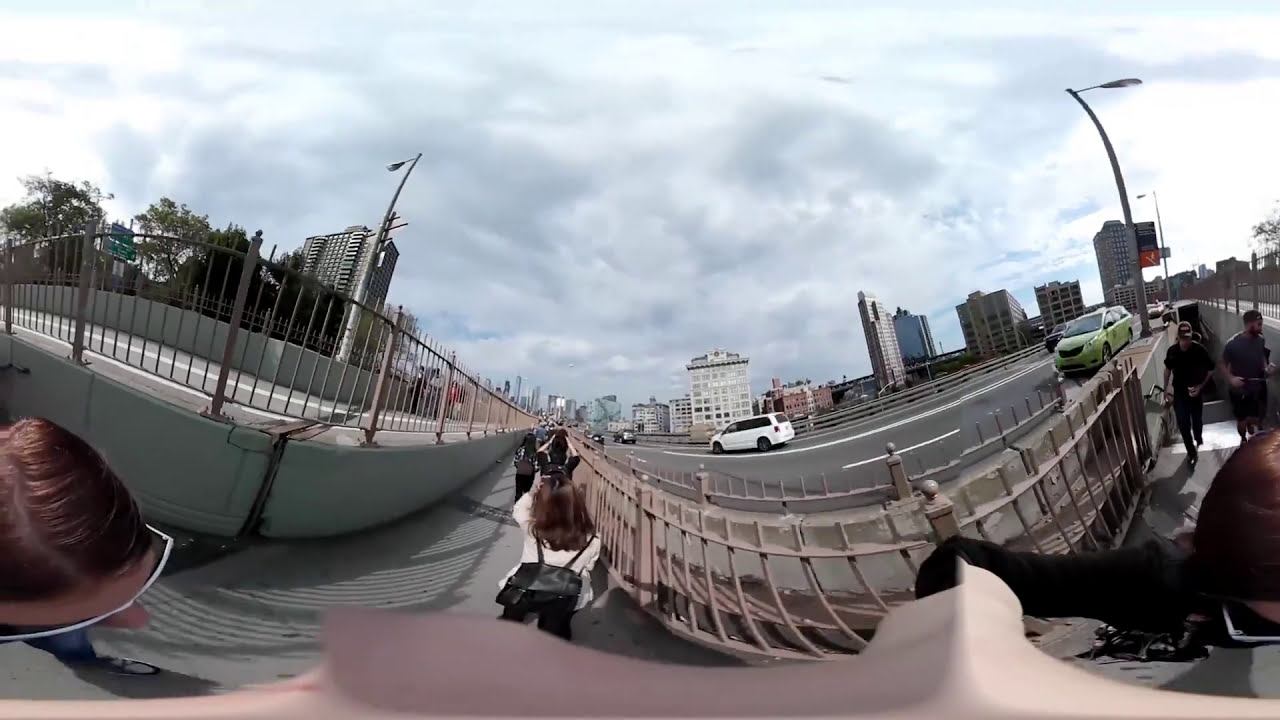The image captures a bustling urban scene from a panoramic perspective, primarily showcasing a central sidewalk where numerous pedestrians are walking away from the camera. To the left, there's another elevated sidewalk with two people walking, lined with trees and backed by a high-rise building. Both sidewalks are adjacent to a major urban road, featuring multiple lanes and several vehicles, including a white car and a light green car. The scene includes two men emerging from a subway station on the right. Surrounding the main walkway, there are numerous office buildings, possibly indicative of a metropolitan area such as Atlanta or Los Angeles. Street lamps dot the area, and a light brown fence separates parts of the sidewalk from the road. The sky is overcast but bright, suggesting it is daytime. A woman with brown hair, wearing a white top and a black backpack, is prominently walking in the foreground to the left. The overall environment is characterized by a mix of greenery, extensive infrastructure, and a dynamic urban atmosphere.